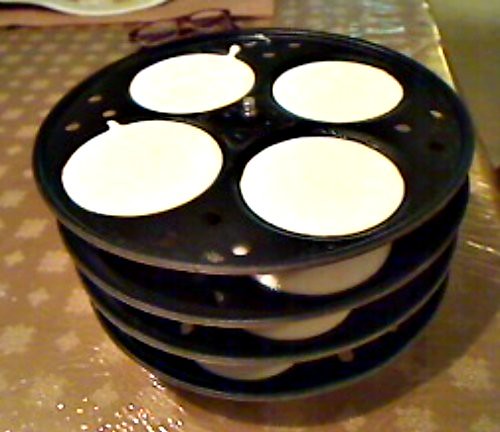This indoor photograph captures a slightly dark, grainy, and out-of-focus scene of a blue linoleum table with light white squares and diamond patterns. In the foreground stands a black, cylindrical rack composed of four perforated layers stacked vertically on a central chrome stem. The topmost rack, clearly visible, contains four evenly spaced pools of white batter, likely pancake or muffin batter. The three lower racks appear to hold cooked contents, which seem puffed up compared to the batter-filled top rack. A pair of reddish, closed reading glasses rests just left of center near the top of the frame, highlighting the domestic setting. At the upper right, the edge of the table can be seen, adding context to the cozy, slightly cluttered scene.